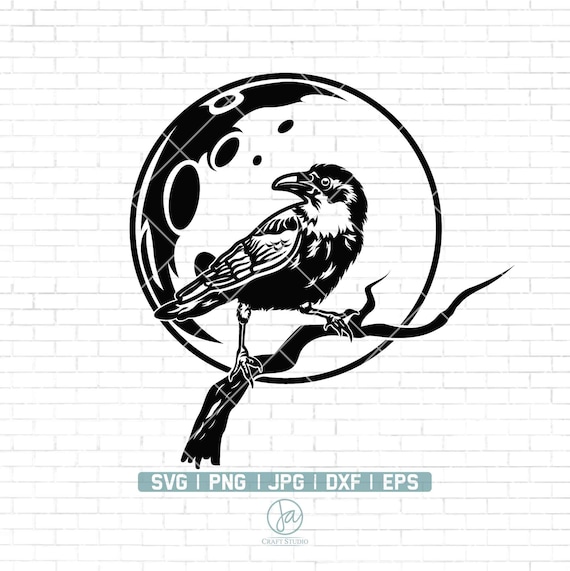The image is an intricate black and white illustration set against a very light gray-green brick background. At the center is a detailed drawing of a crow standing on a tree branch. The crow's body faces right while its head looks back over its shoulder to the left, towards a moon behind it. The moon is depicted with a shaded crescent on the right upper portion and several black craters on the upper left. Surrounding the bird is a circular transparent bubble with dark shading on the left side, suggesting areas of non-transparency. Below this imagery, there is a light teal rectangle containing white text that reads "SVG, PNG, JPG, DXF, EPS". Beneath this, there is a teal circle outlined with the letters "JA" inside, representing Jacraft Studio.